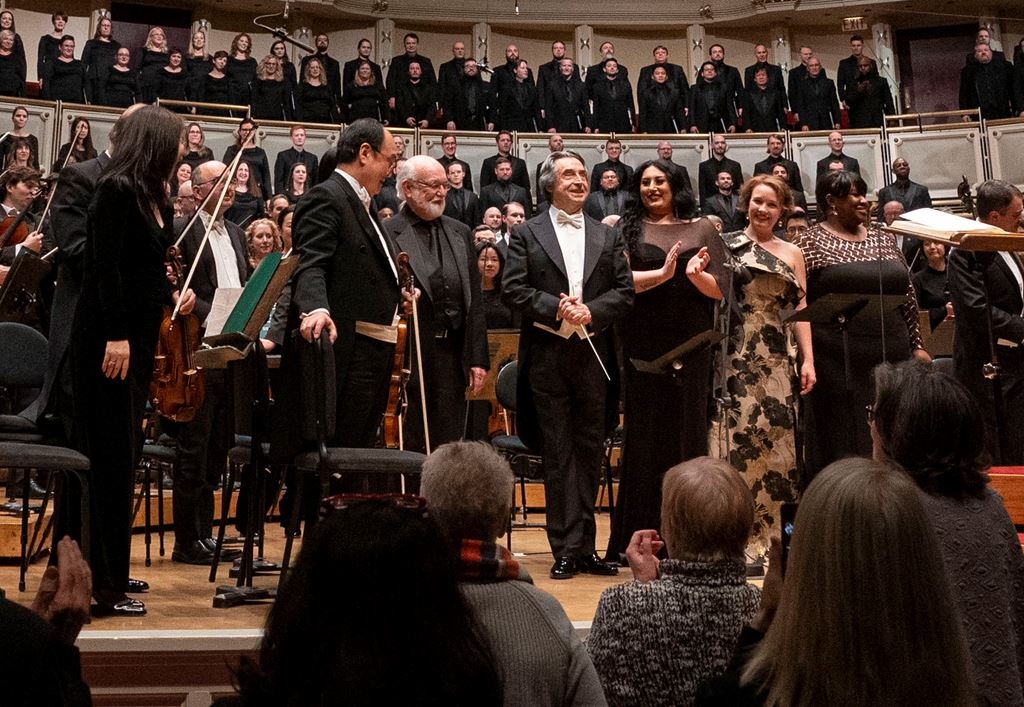The photograph captures an indoor orchestral performance nearing its conclusion, likely inside an opera house or a similar venue. At the forefront of the stage stand three men and four women, with the men donning tuxedos. Among the women, one wears black pants with a black blazer, another a floral dress, and others different black dresses with one having a floral top pattern. The orchestra conductor, an older man in a suit and bow tie, stands prominent with his metal wand, orchestrating amidst applause. To his right is an older man and several women, one of whom claps her hands.

Surrounding this main group, numerous musicians sit or stand, holding instruments like violins and violas, ready to join in acknowledgment. Behind them, an imposing choir arranged in an arc pattern spans four rows. They stand in the balcony, dressed uniformly in black. The audience, visible only by the backs of their heads, applauds enthusiastically, encapsulating the scene in a moment of shared admiration and accomplishment as the performers prepare for their bows.